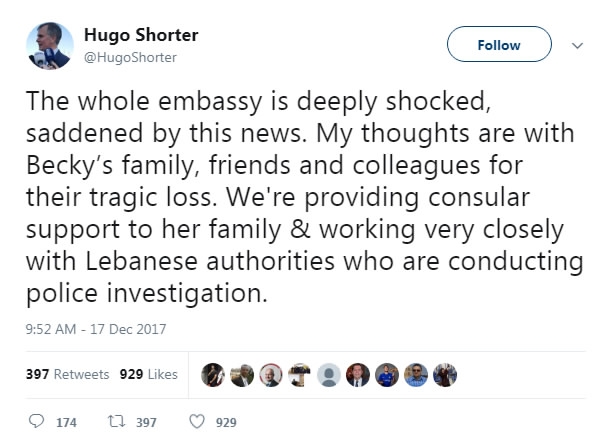In the image, there is a social media post by an individual named Hugo Shorter. The post features a photograph of Hugo Shorter, likely a man based on the image, dressed in a formal suit and a white button-down shirt. He has blackish-gray hair and appears to be making a speech, positioned in front of large media microphones. Hugo is looking to the side as he addresses an audience.

The text accompanying Hugo's image reads: "The whole embassy is deeply shocked and saddened by this news. My thoughts are with Becky's family, friends, and colleagues for their tragic loss. We are providing consular support to her family and working very closely with Lebanese authorities who are conducting a police investigation."

In the upper right corner of the post, there is a white follow button with blue lettering, outlined in blue, accompanied by a gray drop-down arrow. The timestamp on the post indicates it was made at 9:52 a.m. on December 17th, 2017. The post has garnered substantial interaction, with 397 retweets and 929 likes. Additionally, there are profile picture icons of users who interacted with the post, showing about 10 in a row, followed by the number 174. Below this, icons illustrate interactions: a speech bubble representing comments (174), two arrows symbolizing retweets (397), and a heart indicating likes (929).